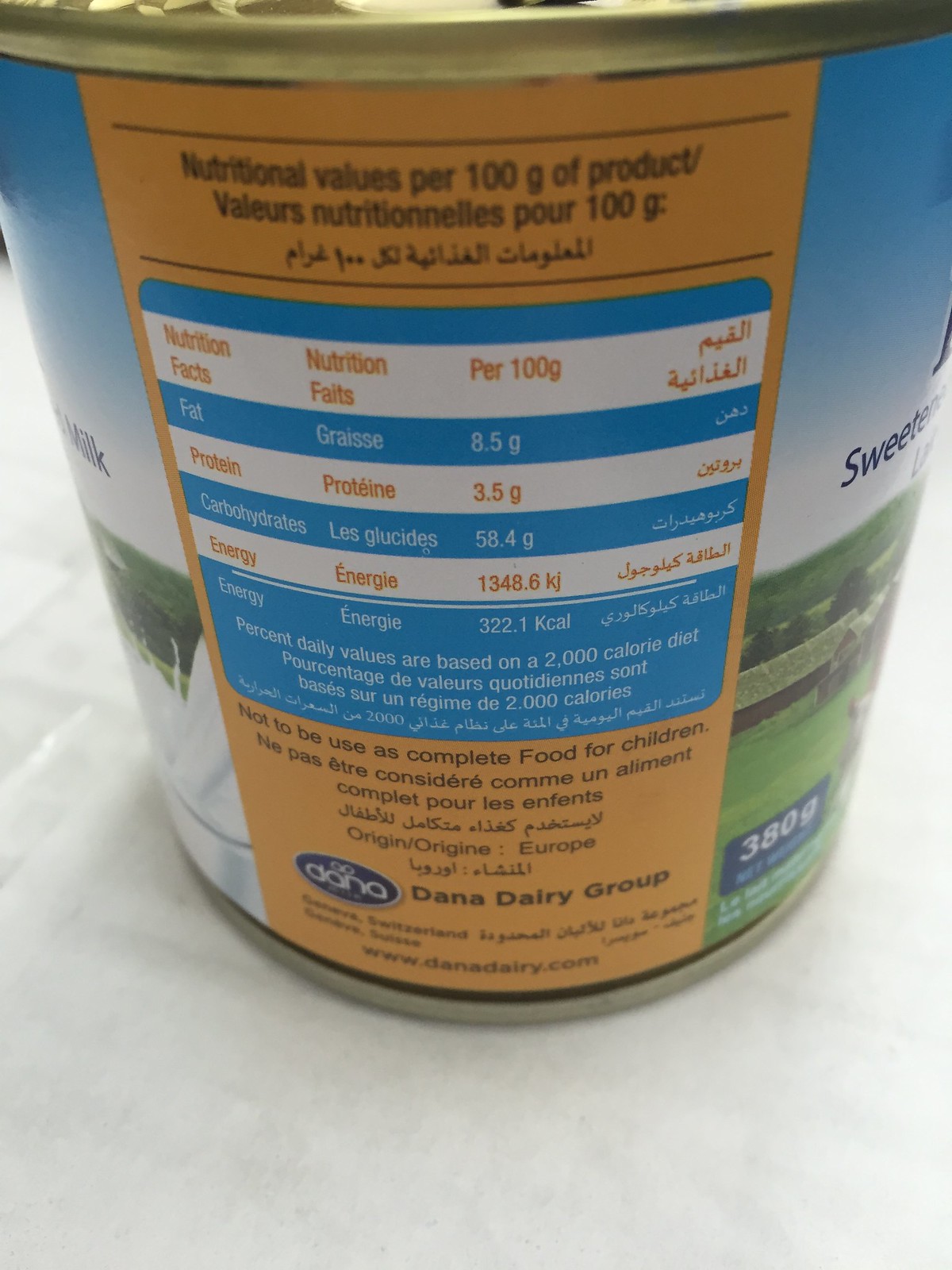The image is a detailed photograph of the nutrition facts label on the back of a yogurt container, which is manufactured by the Dana Dairy Group. The label is predominantly orange with black text, clearly displaying nutritional values per 100 grams of the product. Key nutritional facts include 8.5 grams of fat, 3.5 grams of protein, 58.4 grams of carbohydrates, and an energy value of 1348.6 kJ. The label also notes that the product should not be used as complete food for children. Positioned on a white surface, the container is colorful, depicting a milk product being poured into a clear glass on one side and an idyllic image of a green meadow with cows under a blue sky on the right side. The label indicates that the product weighs 380 grams and features the Dana Dairy Group's blue logo at the bottom. Some information appears to be in a different language.